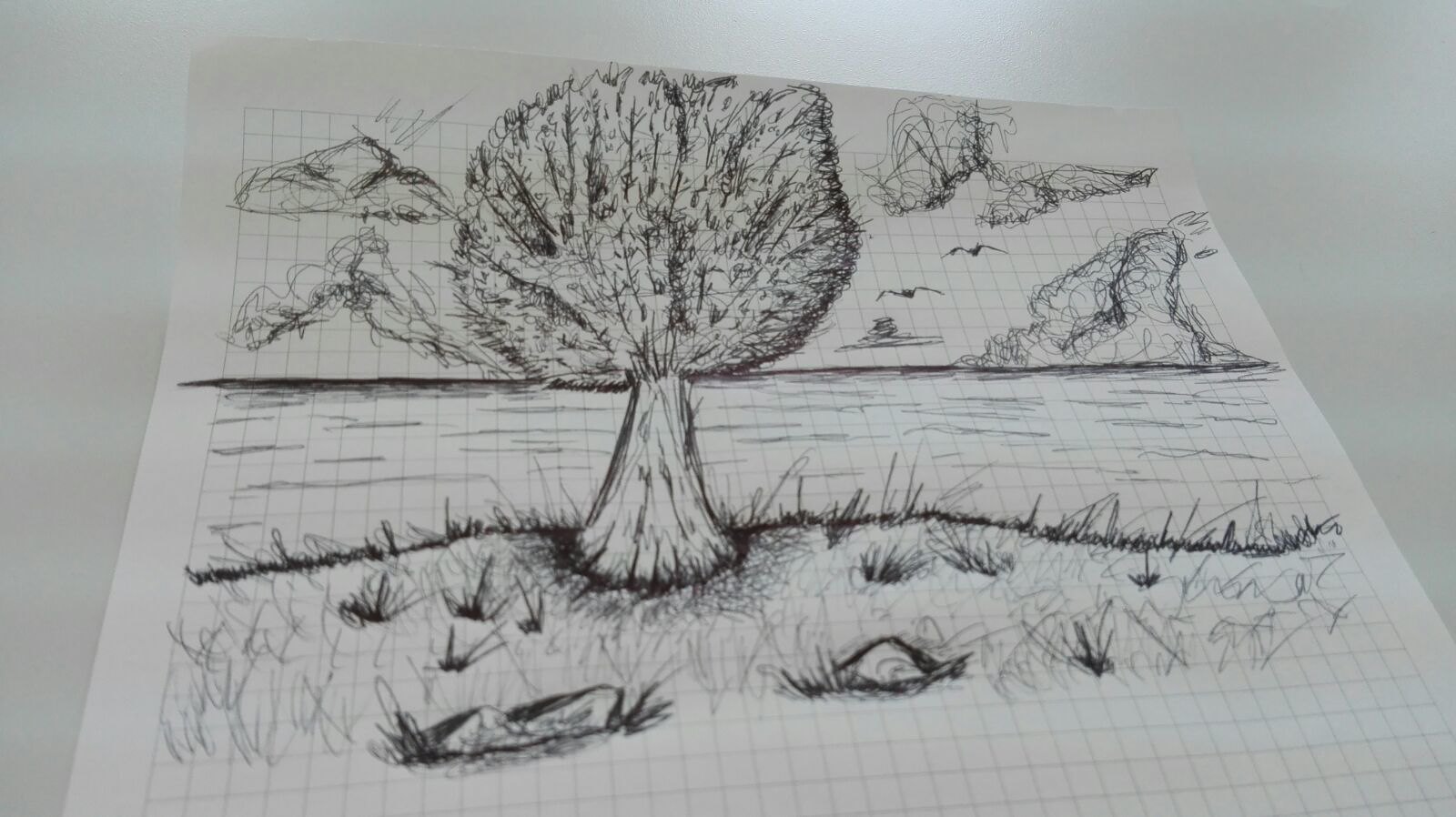The photograph depicts a detailed pen and ink drawing on a piece of white paper, set against a mostly gray countertop or table. Dominating the scene, the white paper contrasts sharply with the gray background, making the artwork stand out. The drawing captures a solitary tree rising from a small patch of sand and grass. The tree features a wide trunk that tapers as it ascends, culminating in a rounded treetop with intricately rendered branches. Surrounding the tree's base, the artist has depicted scattered rocks and tufts of grass, adding texture to the foreground.

In the background, a clear horizon line separates a serene body of water from the sky. The sky itself is adorned with several clouds, illustrated in a whimsical, scribbly style, and complemented by a few birds that add life to the scene. The detailed elements of the drawing, from the intricate tree to the textured ground and dynamic sky, create a rich, engaging visual narrative.